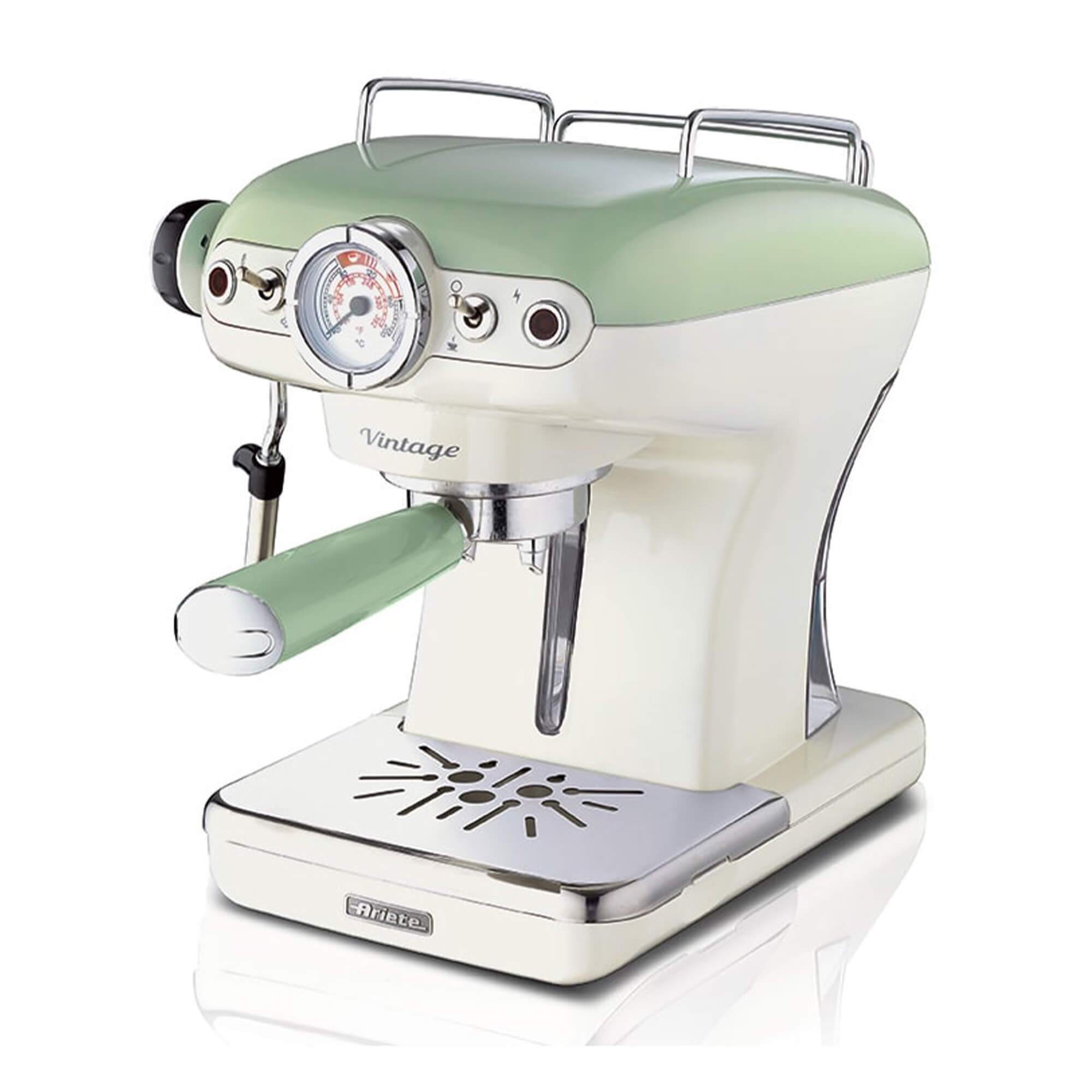This is an image of a vintage-style coffee machine, branded as Ariete. The machine features a cream and mint green color scheme with steel details, emphasizing its retro aesthetic. It has an organic shape that adds to its vintage charm. Central to the machine is a prominent, smooth, polished lever in muted sage green, which likely serves as the handle for the coffee grounds. Above this lever is a circular gauge that possibly indicates temperature or time, situated symmetrically between two indicator lights.

Flanking the central gauge and lights are two control knobs, each marked with numbers for various functions, further contributing to the machine's symmetrical design. However, the machine has a larger turn dial on the left-hand side which slightly disrupts this symmetry. The machine also features a spot intended for placing a mixing bowl or a cup, possibly for brewing purposes. The overall appearance, combined with the use of plastic and metal materials, reinforces the vintage look while suggesting modern functionality.